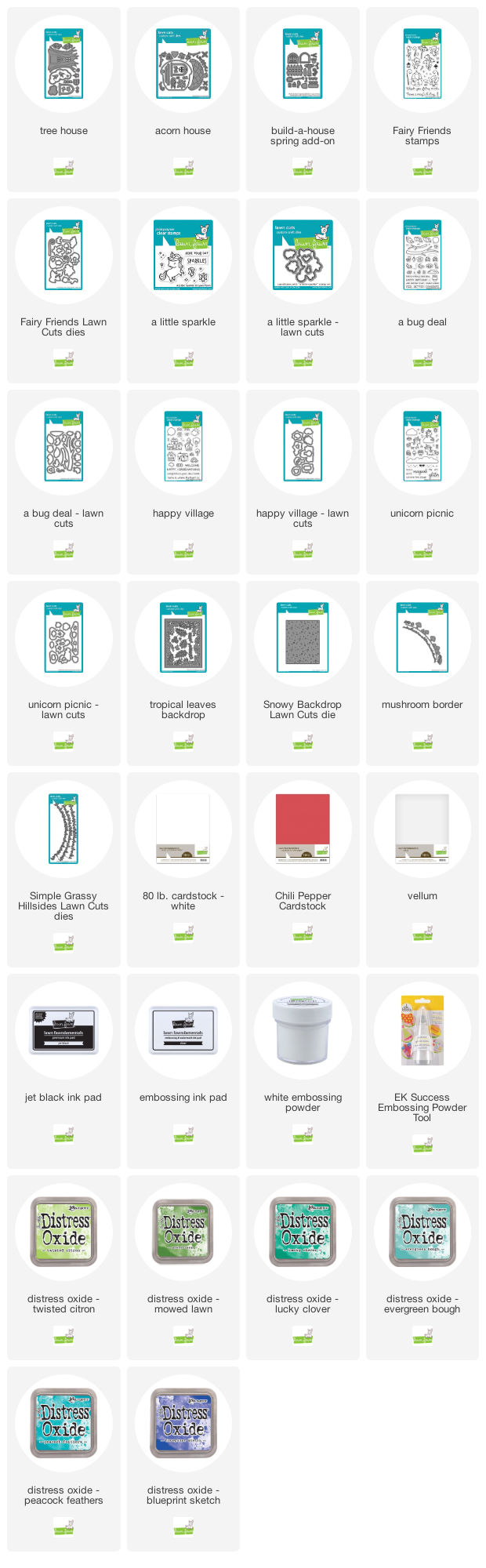The image is a vertically oriented rectangular box displaying a grid composed of 30 smaller rectangles arranged in a structure of four columns and eight rows, although the eighth row contains only two rectangles. Each of these small rectangles features a greenish-turquoise border encompassing an image with a corresponding caption underneath it. Additionally, beneath each caption is a small green emblem, which is consistently present across all the individual rectangles. The images and text appear uniform but are challenging to decipher due to their small size and faint print. The top-left rectangle is labeled "treehouse," followed by various other labels that are difficult to read.